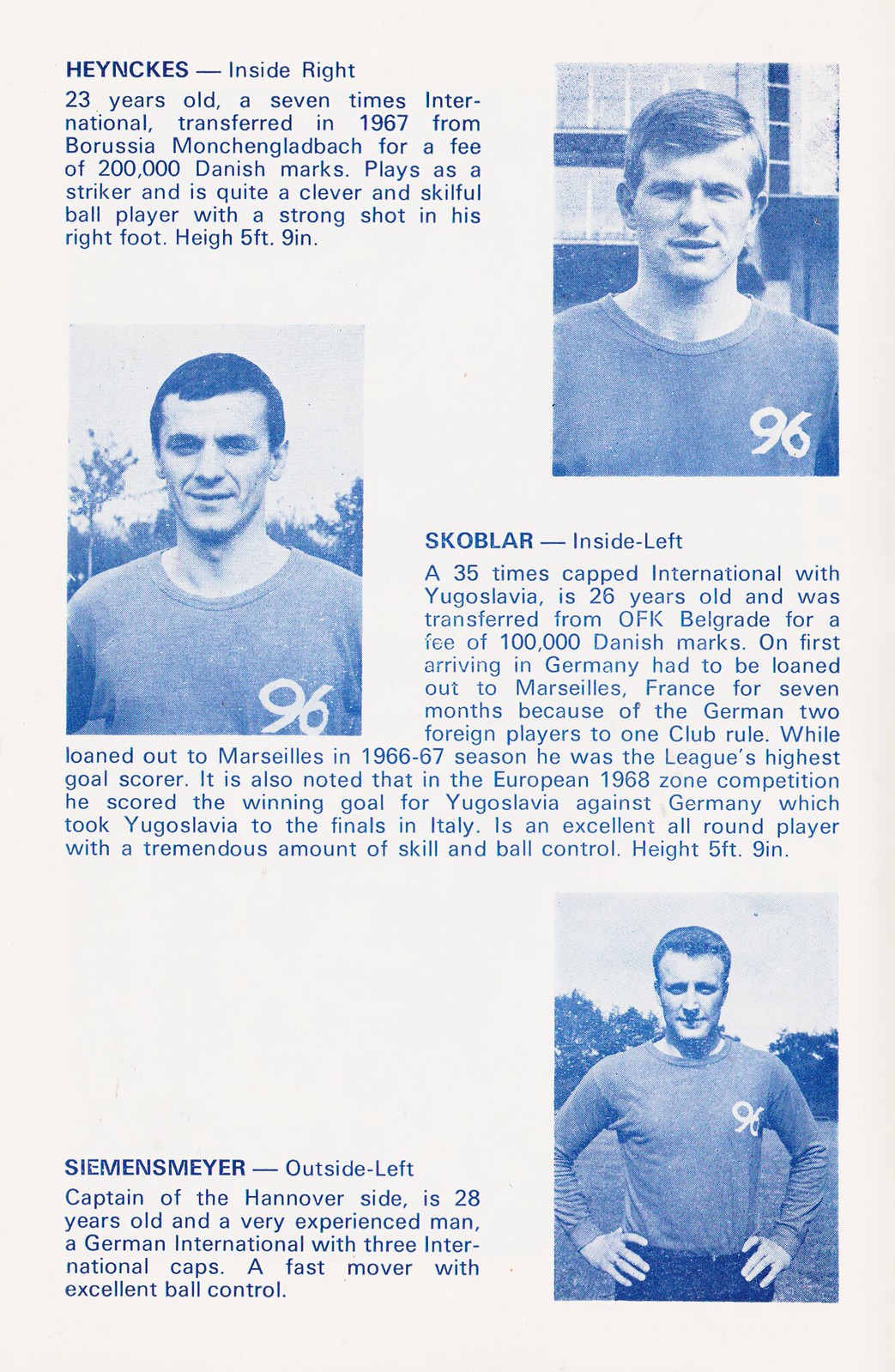The image resembles a vintage page from a sports program, specifically showcasing three monochromatic, blue-and-white photographs of soccer players from 1996. Arranged in a staggered layout with one photo at the top right, the second in the middle left, and the third at the bottom right, each player’s image is accompanied by their name, position, and brief biography.

The first player depicted is Heineke, an inside-right striker, 23 years old, notable for his transfer in 1967 from Borussia Mönchengladbach for a fee of 200,000 Danish marks. Standing 5'9", Heineke is recognized for his clever play and strong right-foot shot, having represented his country seven times internationally.

The second player, Skoblar, positioned at inside-left, is a notable 35-time international captain for Yugoslavia. At 26 years old, Skoblar was transferred from OFK Belgrade for 100,000 Danish marks. Due to the German two-foreign-players-per-club rule, he was loaned to Marseille, where he became the league's top scorer in the 1966/67 season. He is renowned for his skillful ball control and scored the winning goal for Yugoslavia against Germany in the 1968 European zone competition finals.

The third player, Siemsenmeier, is an outside-left and the captain of the Hannover team. At 28 years old, he is an experienced German international with three caps. Known for his speed and excellent ball control, he rounds out this vintage soccer program page celebrating these skilled European players. Each player dons a long-sleeve shirt marked with the number 96 and the year on the left breast, adding a cohesive historical touch to the presentation.